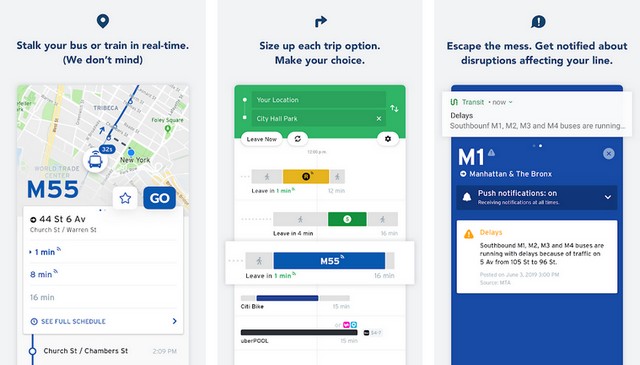**Detailed Caption:**

These vertically oriented images showcase features of a route planning app, potentially indicating its functionality on smartphones. 

1. **Real-Time Tracking and Scheduling:** The first image on the left highlights the app’s real-time tracking capability for buses or trains. It shows the current location of the M55 bus on a miniature map, specifically at the intersection of 44th Street and 6th Avenue. Users are provided with a live update indicating the bus’s arrival in one minute and the next in eight minutes. Additional options include viewing the full schedule, starring the route for quick access, or hitting the "Go" button to plan the journey.

2. **Trip Option Comparison:** The middle image focuses on helping users size up each trip option and make informed choices. The interface has input boxes for the starting point and destination, with the destination pre-filled as "City Hall Park." Users can modify the departure time, with options such as "Leave now" or set a specific time to depart, indicated by options like "Leave in 4 minutes." This section also highlights the M55 bus again, showing an option to leave in five minutes, along with additional trip alternatives below.

3. **Disruption Notifications:** The third panel aims at keeping users informed about delays and disruptions. This screen broadcasts important updates, such as current delays for southbound M1, M2, M3, and M4 buses due to traffic in Manhattan and the Bronx. This feature ensures users receive timely notifications about potential delays affecting their commute, helping them plan alternative routes if necessary.

This comprehensive route planning app appears to be specifically designed for the New York City public transportation system, offering detailed real-time data, customizable trip planning, and disruption alerts.